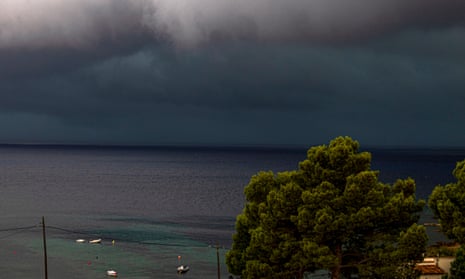The photograph captures a deeply foreboding scene of an approaching storm over the ocean, under a nearly black sky. Dark, tumultuous clouds fill the horizon, contrasting sharply with slight lightness closer to the camera. The ocean itself appears menacing with its dark purple and blue hues, yet retains a deceptive calmness. In the waters, several small white boats, including two with little flags, are visible, potentially hinting at life amidst the impending chaos. The bottom right corner of the image reveals tall green trees, suggesting late summer, and the hint of a house with lights on, partially obscured by the foliage. To the bottom left, a few power lines run parallel to the tops of the trees, intersecting the composition. The overall scene evokes a strong sense of anticipation and artistic tension, capturing the raw power of nature and the subtle presence of human life.